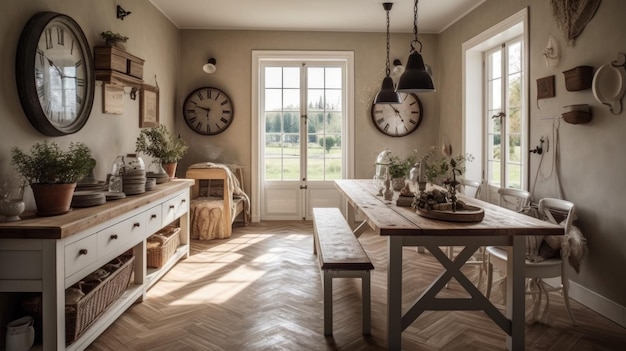The image depicts a cozy kitchen dining area with a country living vibe. The walls are beige with tall white baseboards, creating a warm yet clean look. On the right side of the image, there's a large window or possibly a glass door framed in white, offering a glimpse of the outside with grass, trees, and a cloudy gray sky.

Centrally positioned on the far wall are two narrow rectangular doors, also framed in white, likely leading to the outside. The room is filled with natural light shining through these openings. Flanking these doors on both sides are large, round clocks, white with black frames, adding symmetry and a rustic charm.

To the left, a matching large round clock adorns the wall above a long white cabinet with a wooden top. This cabinet features multiple drawers, a bottom shelf, and is decorated with several potted plants in terracotta pots, enhancing the room's inviting atmosphere. Below the cabinet, wicker baskets add to the storage solutions while maintaining the room's aesthetic.

The dining area features a large picnic-style table with a natural wood tabletop and white base. On one side of the table is a wooden bench, while the other side is furnished with two white chairs. More potted plants and plates are placed on the table, completing the setup. The floor beneath is a zigzag pattern of light hardwood planks, contributing to the cozy, rustic feel of the room.